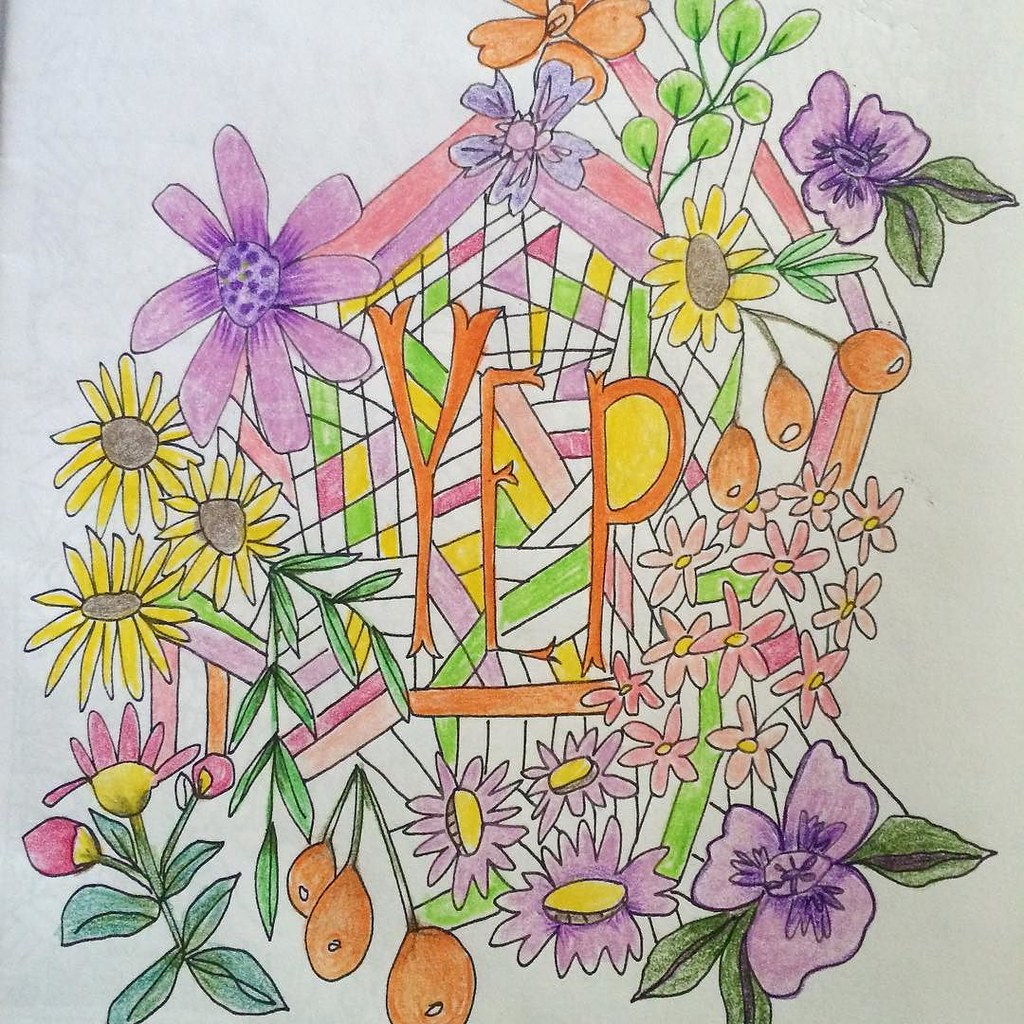The artwork depicts a serene and delicate composition of flowers and fruit rendered in soft, pastel hues with colored pencils. Various flowers in shades of violet and pink gracefully intermingle, some showcasing vibrant yellow centers that draw the eye. At the bottom of the piece, clusters of small, orange fruits dangle, adding a touch of warmth to the scene. The heart of the drawing is marked by three letters, 'Y-E-P,' subtly outlined in a gentle orange, with the 'P' having a bright yellow center. This tranquil arrangement evokes feelings of peace and joy, capturing the harmonious beauty of nature with understated elegance.